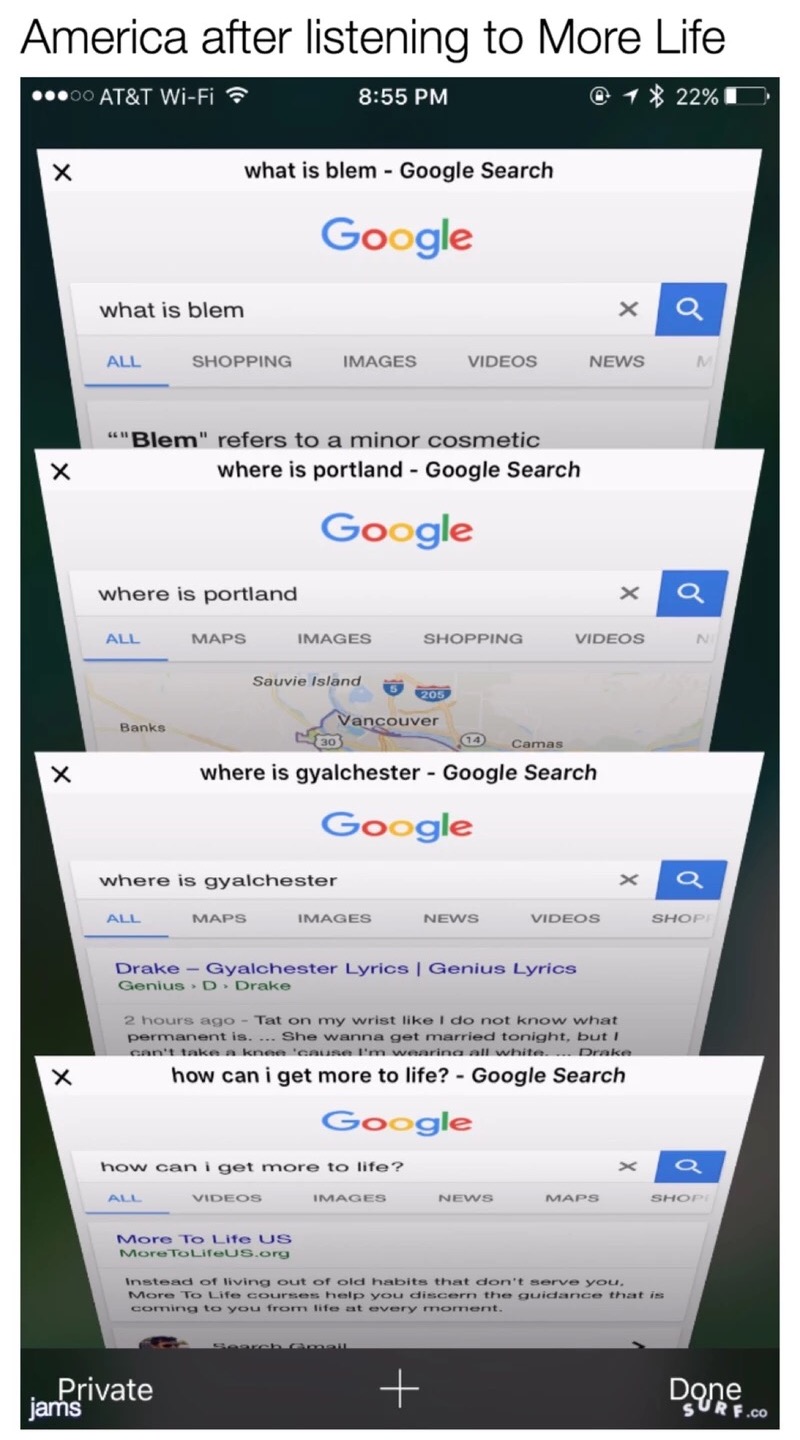This is a detailed caption for the described image:

A screenshot captured from an iPhone shows various snippets of information and a few searches in the Safari web browser. The text at the very top reads "America after listening to More Life." The status bar at the top indicates that the device is connected to AT&T Wi-Fi, the time is 8:55 PM, and the battery is at 22%.

The screenshot displays four tabs open in Safari:

1. The first tab is a Google search for "what is BLEM." Visible text mentions that "BLEM refers to a minor cosmetic," but the full explanation is cut off.
2. The second tab features a search for "where is Portland," displaying a map highlighting the Portland area and parts of Vancouver in either Oregon or Washington.
3. The third tab is another Google search for "where is Galchester," with visible search results including a link to Genius Lyrics related to the song "Glychester" by Drake.
4. The fourth tab queries "how can I get more to life," with a visible result from a website named moretolifeus.org.